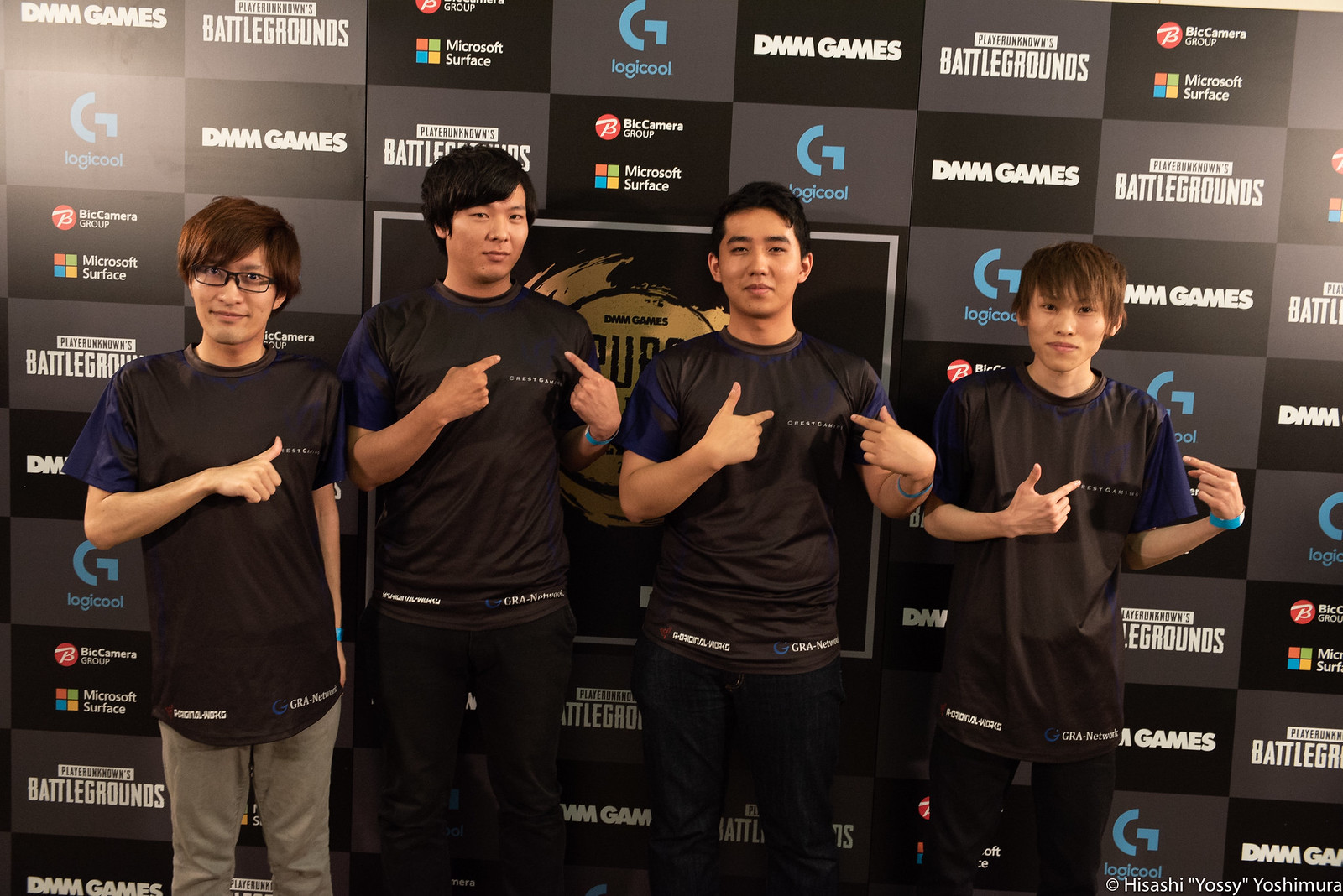The image features four young Asian males standing in front of a backdrop adorned with various game company logos, including Microsoft Surface, Logicool, Big Camera Group, DMM Games, and PlayerUnknown's Battlegrounds, all repeated in black and gray squares. They are identically dressed in black t-shirts with blue sleeves and black pants, except for the man on the left who is wearing gray pants. Each is pointing to a "Crest Gaming" logo on their shirts, which also feature additional logos near the hem, such as "GRE Network." The setting appears to be a professional or promotional event, likely related to gaming or eSports, given the prominent sponsor branding in the background.